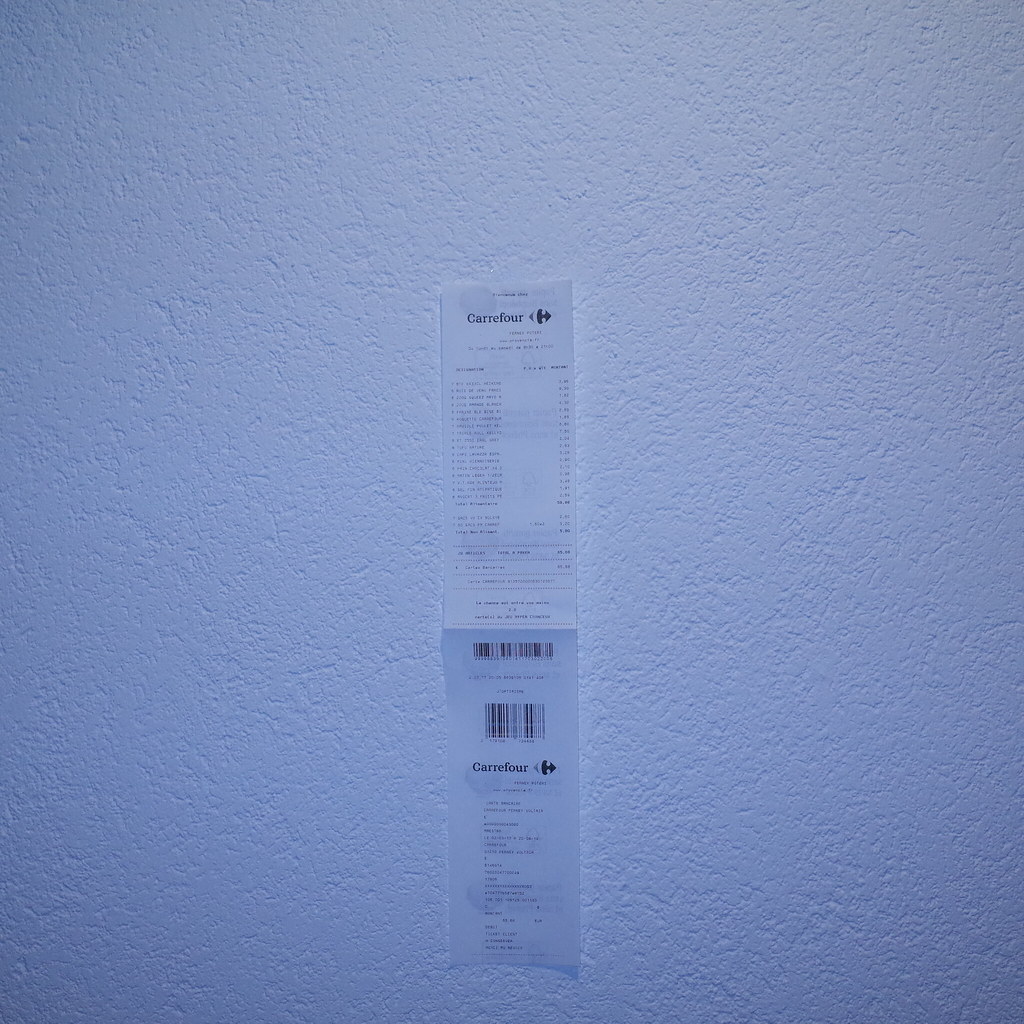A long receipt from Carrefour is affixed to a white wall, stretching from slightly above the center of the wall down to its base, nearly reaching the bottom of the photo. At the top of the receipt, the store name "Carrefour" is prominently displayed. Beneath this, there is a densely packed list of purchased items, printed in such small text that it is barely legible. Further down the receipt, two barcodes are visible—one positioned above the other. Toward the bottom of the receipt, the store name "Carrefour" appears once again, followed by a cluster of additional text rendered in similarly tiny letters, making them indistinguishable from a distance.